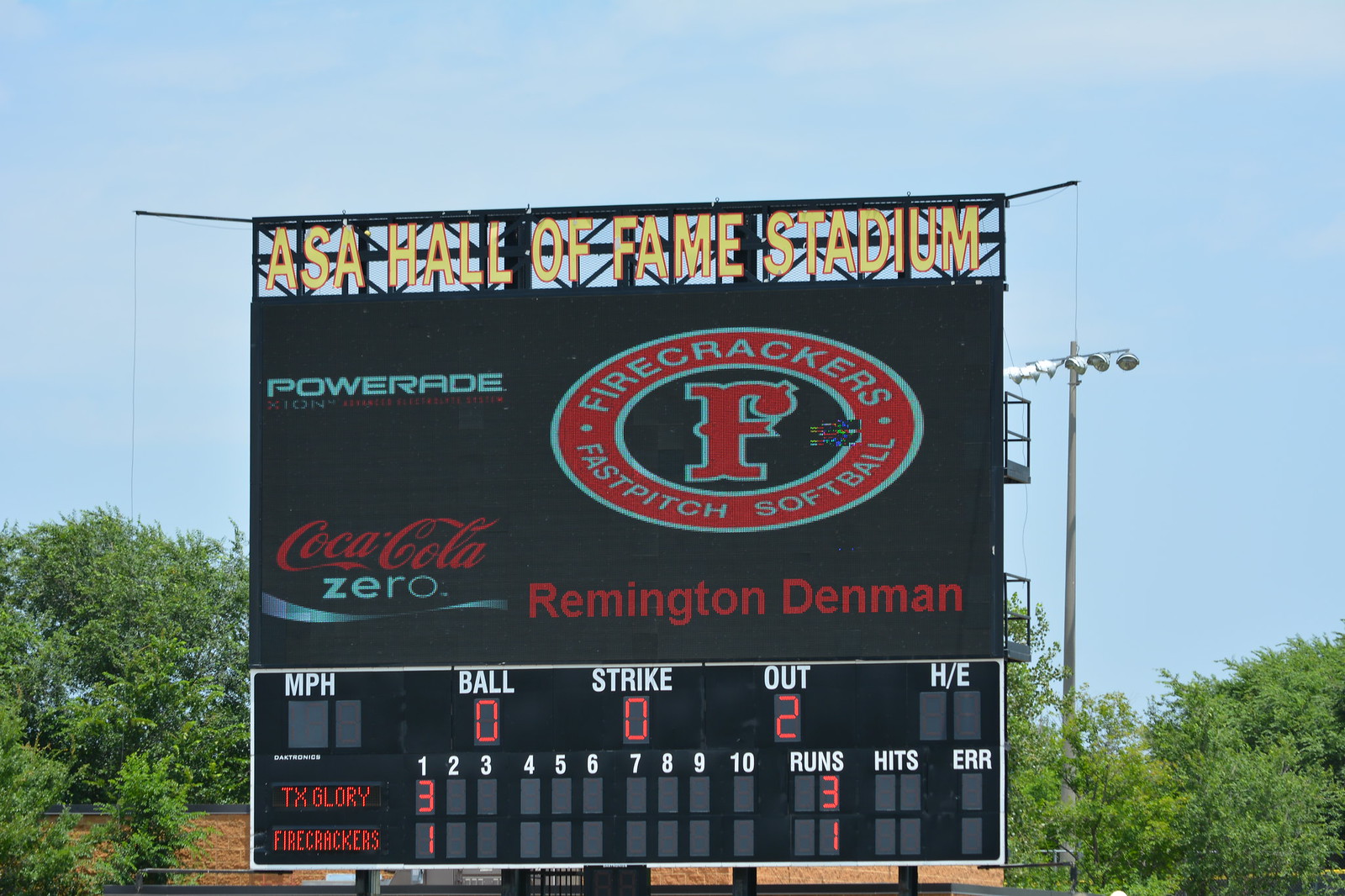The image captures an outdoor scene centered around a large, black baseball scoreboard located at the ASA Hall of Fame Stadium. The top of the scoreboard prominently displays "ASA Hall of Fame Stadium" beneath which the words "Powerade" and "Coca-Cola Zero" appear on screen displays. To the right of these, there's a logo with a red "F" that reads "Firecrackers Fast Pitch Softball" followed by "Remington Denman." 

Below these logos, the conventional baseball scoreboard shows details such as "MPH," "Ball," "Strike," "Out," and "H/E." At this moment, the board indicates it is the first inning with TX Glory leading the game with three points against Firecrackers’ one. The count shows zero balls, zero strikes, and two outs. 

Surrounding the scoreboard, the background features a clear, blue sky with some white clouds and green trees, enhancing the outdoor, daytime setting. The natural light vividly illuminates the robust black structure against the serene sky, creating a bright and clear image.